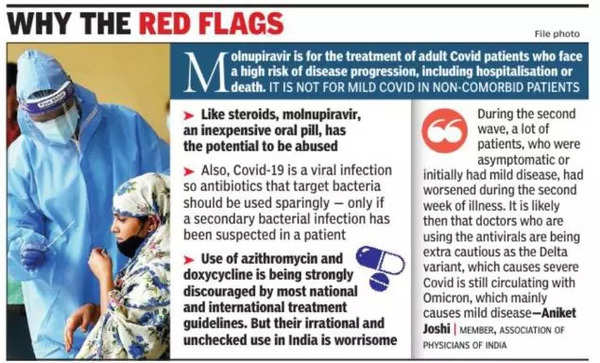Caption: 

The image shows a detailed news article titled "Why the Red Flags". On the left side of the image, a person is dressed in a full blue hazmat suit and visor, standing beside a seated figure who appears to be ill. The seated person is covered with a floral-designed blanket over their head. 

The article discusses the use of Molnupiravir, an oral antiviral medication, for the treatment of adult COVID-19 patients at high risk of severe disease progression. It is not recommended for patients with mild COVID-19 who have no underlying health conditions. The potential for misuse of Molnupiravir, similar to steroids, is highlighted due to its affordability and ease of use. Additionally, the article stresses the appropriate use of antibiotics, which should only be administered if a secondary bacterial infection is suspected, as COVID-19 is caused by a virus. 

On the right, there is a quote by Aniket Joshi, a member of the Association of Physicians of India, discussing the cautious use of antivirals during the second wave of COVID-19. This wave saw many asymptomatic or mildly affected patients develop severe symptoms in the second week of illness, compounded by the circulation of the Delta and Omicron variants.

The information underscores the complexities and cautious approaches required in treating varying severities of COVID-19 during the ongoing pandemic.